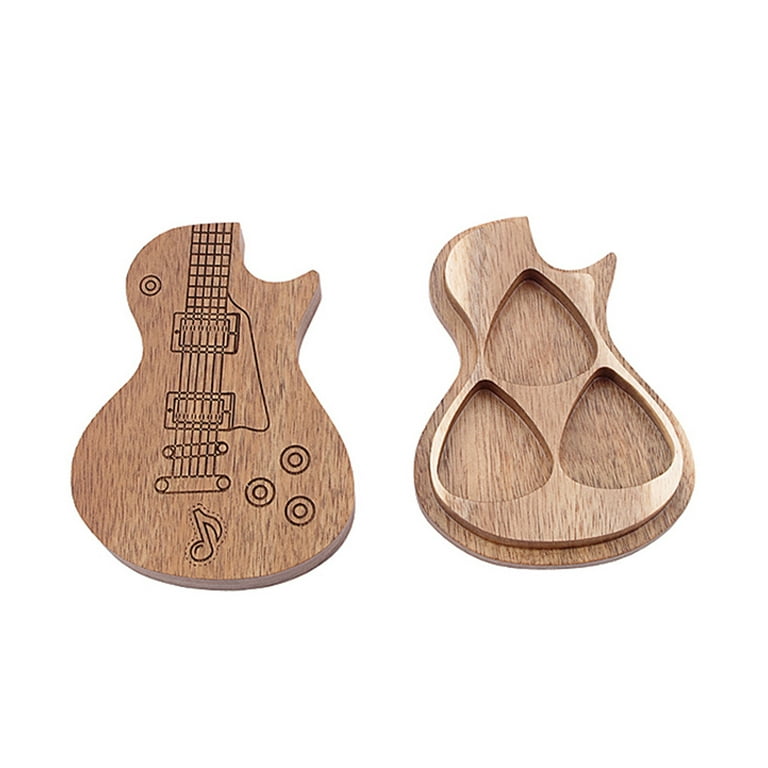The image showcases a wooden guitar pick box designed in the shape of an electric guitar against a solid white background. The box is divided into two parts: the top cover is on the left and the bottom container is on the right. The top cover, crafted from light-colored wood, displays a simple line drawing that accurately depicts various parts of an electric guitar, including the knobs, strings, frets, and the bottom base. This intricate design highlights the attention to detail and the natural wood grain of the material. The bottom half of the box, also wooden, features three compartments carved in the shape of guitar picks, arranged to form an upward-facing triangle. The edges of the bottom part are raised slightly, forming a lip to secure the cover in place. The interior of the bottom half appears to have a glossy finish, emphasizing the wood's texture and providing a smooth surface to hold the guitar picks.